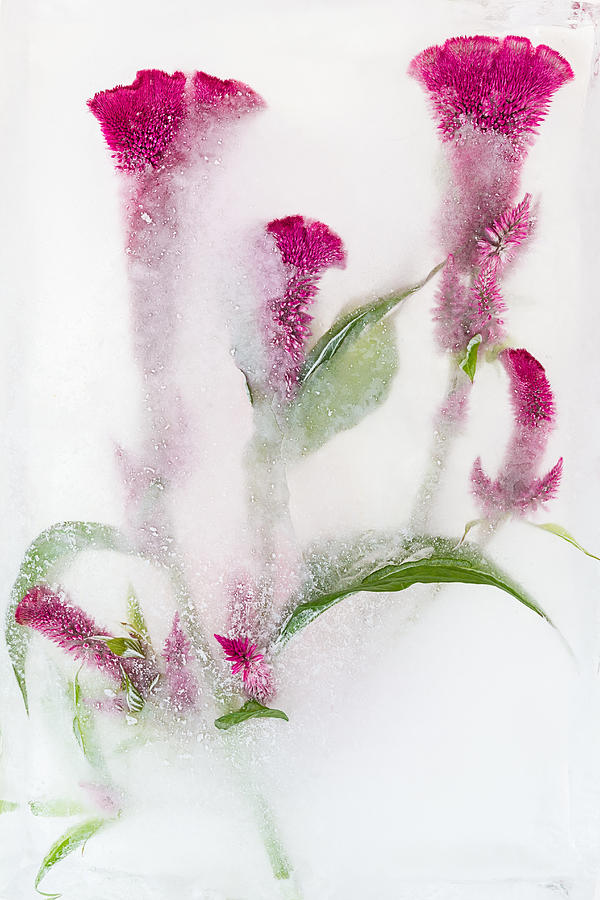This striking image showcases a flowering plant in full bloom, with both bright red and purple elongated flowers emanating from a backdrop of lush green foliage. The plant appears to be engulfed in a mysterious and ethereal white substance, which could resemble frost, snow, or even a translucent layer of ice, adding an intriguing visual element. The vivid colors of the flowers and leaves pop vividly against this white, smoky backdrop, creating a mesmerizing contrast. Some petals seem to break free through the frosty shroud, as if emerging from ice, accentuating the frozen-in-time effect. The overall scene is both beautiful and enigmatic, blending elements of nature with a touch of whimsy.